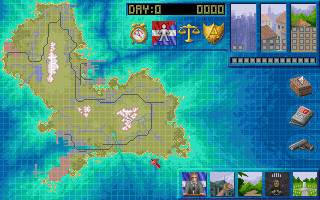Screenshot from a video game showing "Day Zero" with a score of zero points prominently displayed in the center. The background features a detailed map of an island, which is divided into several sections. The island landscape is lush and green with various natural features such as rivers, lakes, and mountains. Surrounding the island, the ocean transitions from green to blue hues. Additionally, the screenshot includes small individual icons or shots, presumably representing different levels, tasks, or hikes that a player can choose from. The interface suggests an open-world exploration game with various objectives to accomplish.